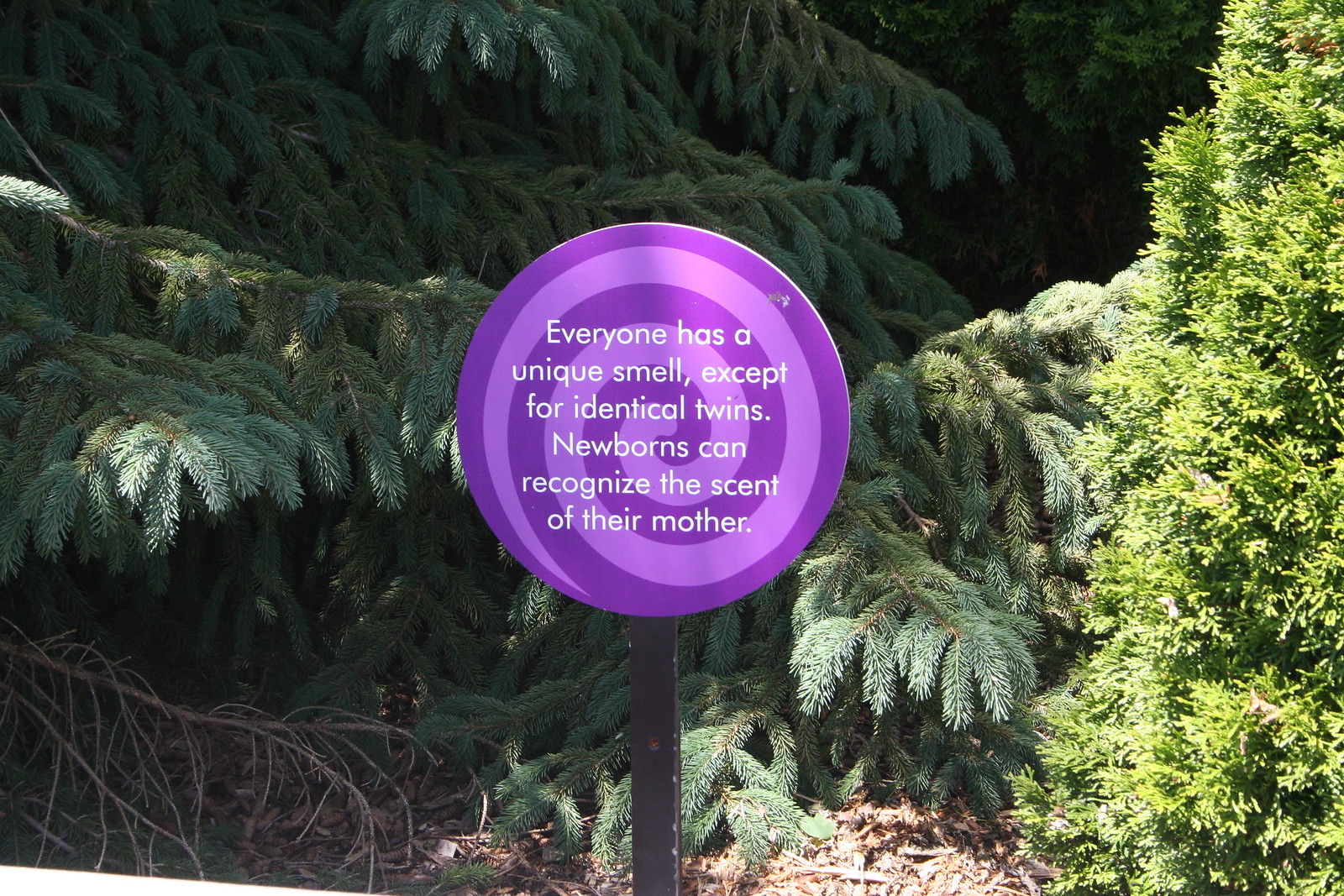The photograph captures a round sign with a striking purple and lilac spiral design, overlaid with white text stating: "Everyone has a unique smell except for identical twins. Newborns can recognize the scent of their mother." This sign is mounted on a dark wooden post. The background features a densely forested area with various pine and fir trees. The branches, laden with green needles, stretch down to the forest floor. Among the trees, a bush or tree without flowers and some bare branches are also visible. The ground beneath the sign is covered in mulch and patches of dirt. Overall, the image presents a serene and natural woodland setting where the sign stands out prominently amidst the greenery.